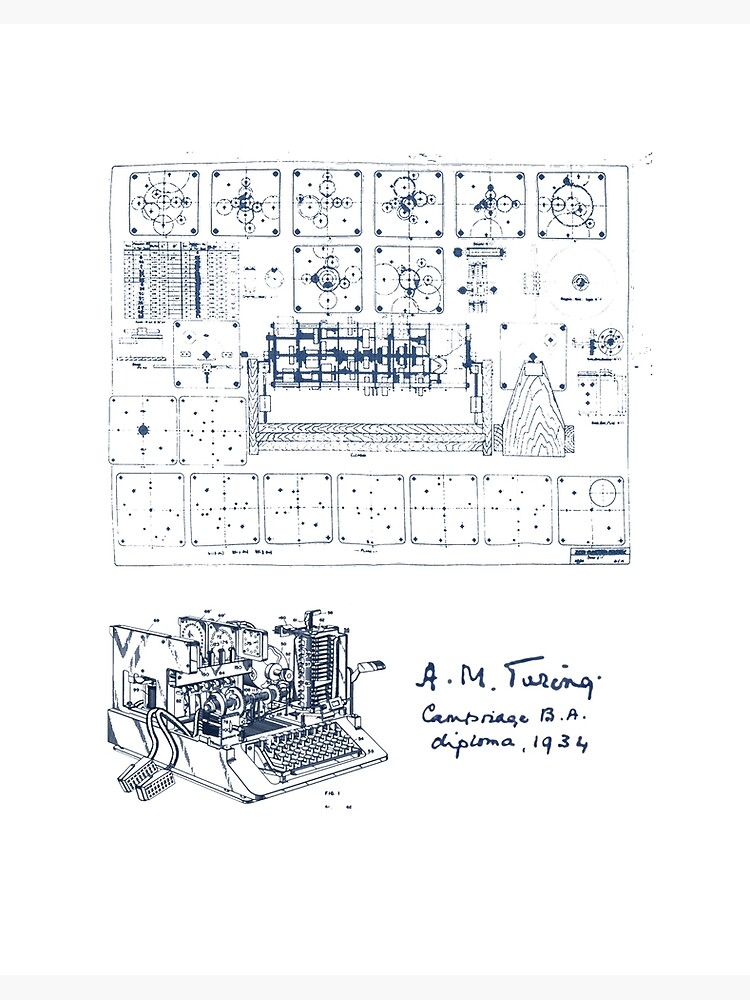The image displays a detailed technical blueprint of a complex machine, seemingly a typewriter, with its intricate inner workings exposed. The blueprint is densely populated with gears, poles, and other mechanical components, revealing the sophisticated design of the machine. In the lower left corner, there is an actual image of the typewriter, showcasing its keys and confirming its identity. Above this image, the blueprint comprises numerous small rectangular sections, each containing concentric circles depicting various components of the typewriter. In the lower right, there is text written in blue ink that reads "A.M. Turing, Cambridge, B.A. Diploma, 1934," suggesting the blueprint's provenance and association with the famous mathematician and inventor, Alan Turing.